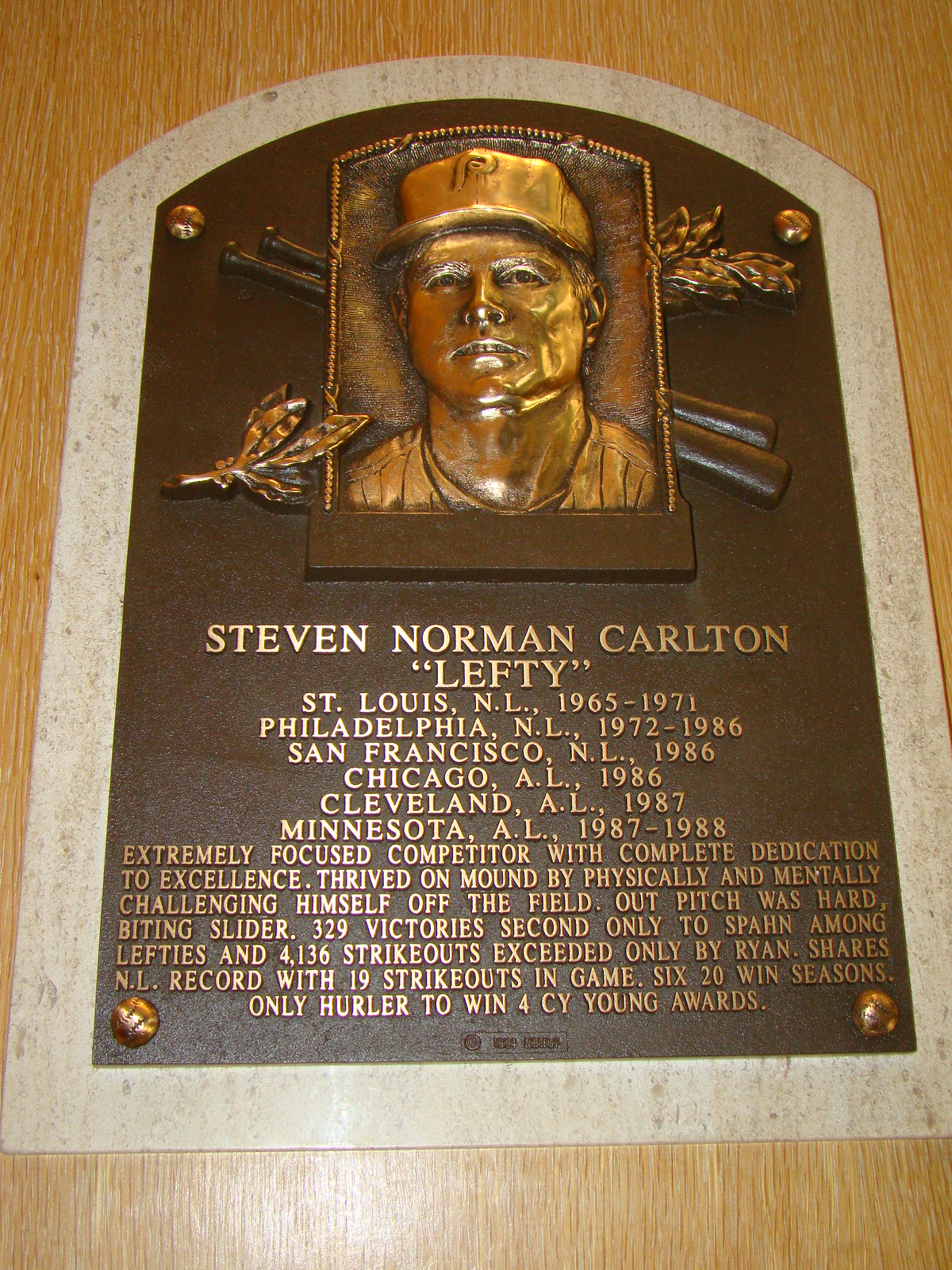This color photograph captures a commemorative plaque mounted on a wood grain wall, presented in portrait orientation with an arched top. The plaque features a dark brown background with gold raised lettering and imagery. At the top center, a golden engraving depicts a smiling baseball player wearing a cap and uniform, with two baseball bats and a flourish of leaves forming an X behind him. The entire top section is bordered with a patterned design.

Secured at each of the four corners by gold baseball-shaped mounts, the plaque honors Stephen Norman "Lefty" Carlton. His career timeline is detailed below his name: 

- St. Louis NL, 1965-1971
- Philadelphia NL, 1972-1986
- San Francisco NL, 1986
- Chicago AL, 1986
- Cleveland AL, 1987
- Minnesota AL, 1987-1988

The inscription commemorates his achievements, noting, "Extremely focused competitor with complete dedication to excellence. Thrived on mound by physically and mentally challenging himself on the field. Out pitch was hard, biting slider... 329 victories second only to Span among lefties and 4,136 strikeouts exceeded only by Ryan. Shares NL record with 19 strikeouts in a game. Six 20-win seasons. One hurler to win four Cy Young Awards." The detailed accolade emphasizes Carlton's distinguished career and notable records in Major League Baseball.